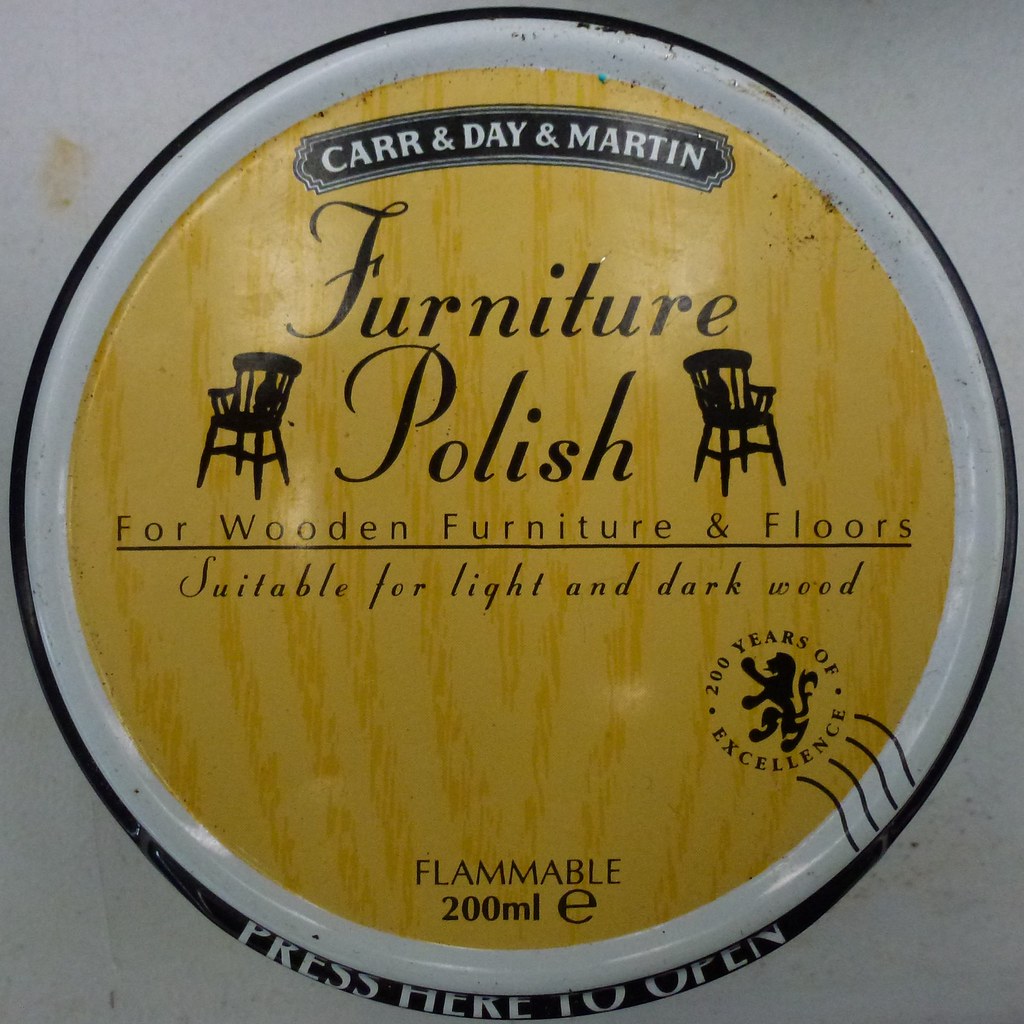This image shows the top lid of a circular container designed to resemble a wooden grain with a yellow and brown textured finish. The container top prominently features a black banner at the top with the words "Carr and Day and Martin" in white text. Below this banner, in an elegant font, it reads "Furniture Polish," flanked on either side by a small black chair illustration. Further down, the text "For Wooden Furniture and Floors" is underlined, followed by "Suitable for Light and Dark Wood" in smaller print. In the lower right corner, there is an emblem of a lion accompanied by the phrase "20 Years of Excellence" circled around it. At the bottom center of the lid, it says "Flammable 200 milliliters." The black border surrounding the lid includes the instruction "Press here to open" at the bottom. The lid rests on a white surface, visible at the corners of the image.